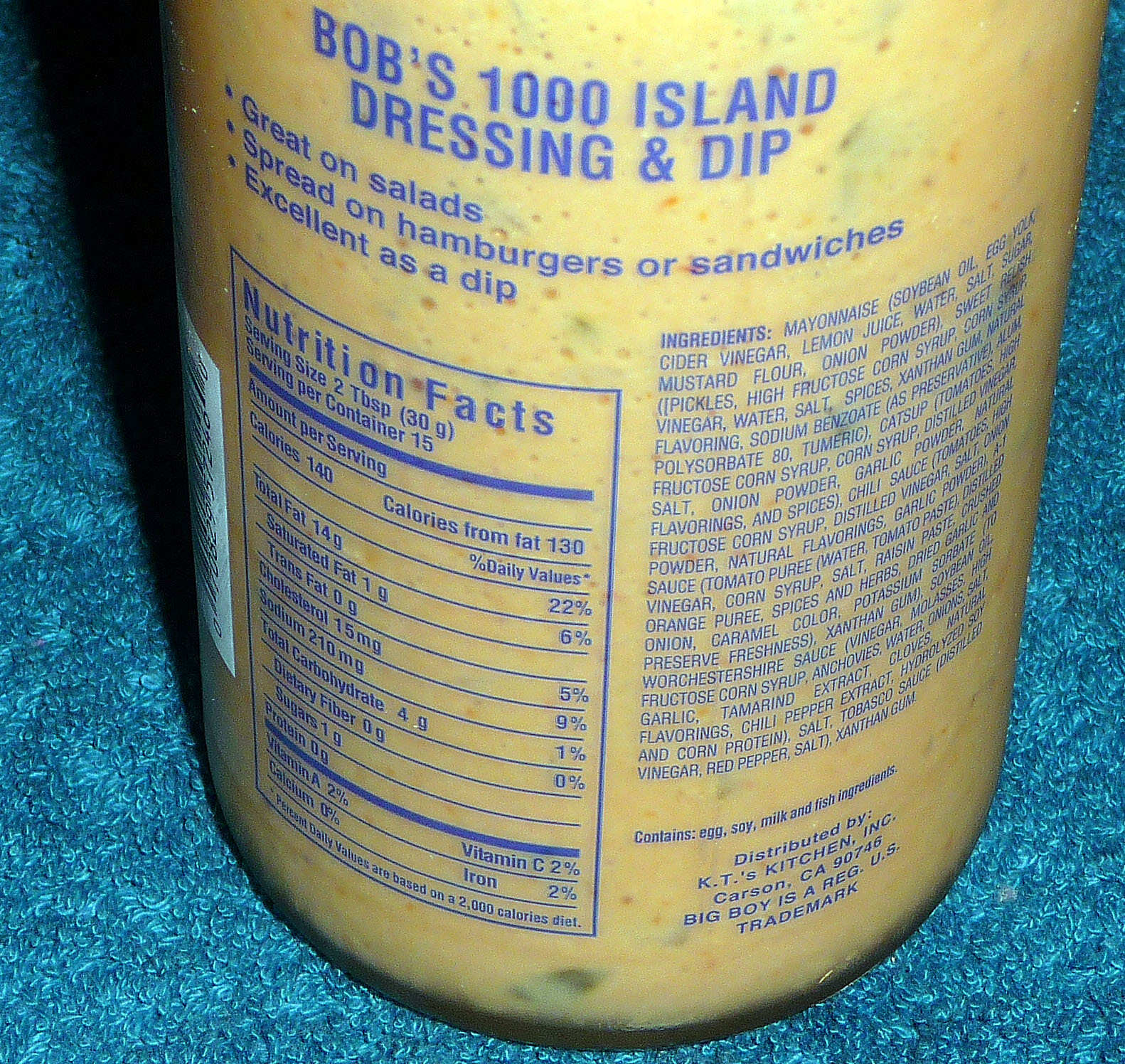The image features a clear bottle of Bob's Thousand Island Dressing and Dip, positioned on a teal, fibrous-textured background that resembles a short carpet or towel. The bottle, captured with a flash, has an orangey-yellow liquid with green flecks, indicating pickles and spices. The label, written predominantly in blue or purple, prominently reads "Bob's 1000 Island Dressing and Dip" and touts its versatility: "Great on salads, spread on hamburgers or sandwiches, excellent as a dip." The left side of the label displays the nutritional facts, while the right side lists the ingredients and dietary warnings, noting it contains eggs, soy, milk, and fish ingredients. Additionally, the label includes the distributor information: KT's Kitchen, Inc., Carson, California, 90746, and mentions that Big Boy is a registered U.S. trademark. The bottle is viewed from a diagonal, slightly top-down angle, which accentuates the shadowing on the left side.